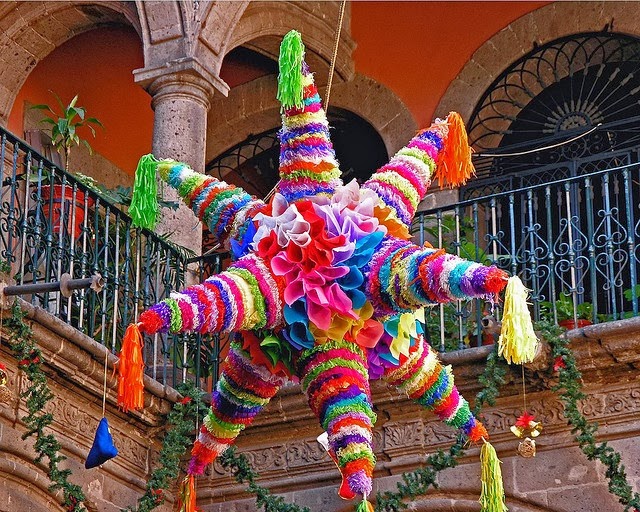The photograph captures a vibrantly colored, traditional star-shaped piñata suspended from the ceiling in the foreground, drawing focus as it dangles vividly against a striking backdrop. The piñata features eight cylindrical cone points radiating from its spherical center, each adorned with vertical stripes in bright hues of yellow, purple, lime green, pink, blue, and dark red, and ending in long, colorful tassels. Surrounding the piñata are ruffled flower shapes made from crepe paper in a spectrum of white, red, pink, purple, and blue.

The scene is set in an open-air courtyard, framed by the upper story of a Spanish-style building. The building's architecture includes beautifully crafted brown Moroccan brick archways and red clay walls with decorative stone pillars. These arches appear along the upper half of the photograph, while below, a black wrought iron balcony hints at the first floor's presence, partially visible with green ivy or garland embellishing the stone cornice.

The overall composition emphasizes the piñata's brilliant colors, contrasting sharply with the muted tones of the brown brick, black iron fencing, and red clay walls. This celebratory element, suspended above the courtyard and centered in the image, appears to float in vivid detail against the rustic and elegant structural elements of the building, evoking a sense of festivity and charm in the setting.